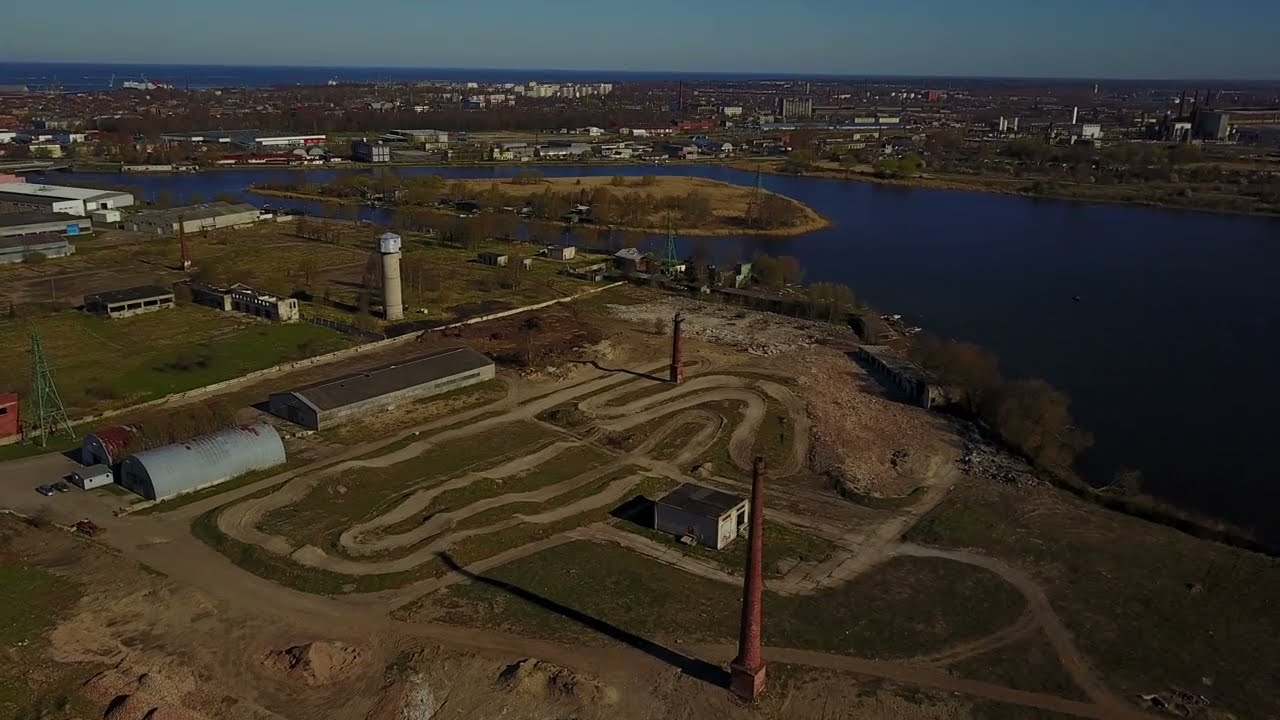In this slightly dark-filtered aerial shot, we see a seafront industrial farmland bordering a calm ocean at the upper portion of the photo. A roadway runs across the center, possibly leading to the distant city visible about two miles away. The bottom half of the image is dominated by sprawling industrial structures, including long barn-like buildings, factories, and hangars, interspersed with patches of green grass and trees. Notably, there are cars parked in the lower left, adding to the sense of a busy, functional area. A small, four-story rectangular building stands out among the mainly two-story structures. The image hints a possible military base or a highly-organized industrial area with barracks and Quonset huts in the top left. A bridge, appearing as a small line due to the aerial perspective, connects two land areas across the water. The dim lighting suggests the photo was taken near dusk.